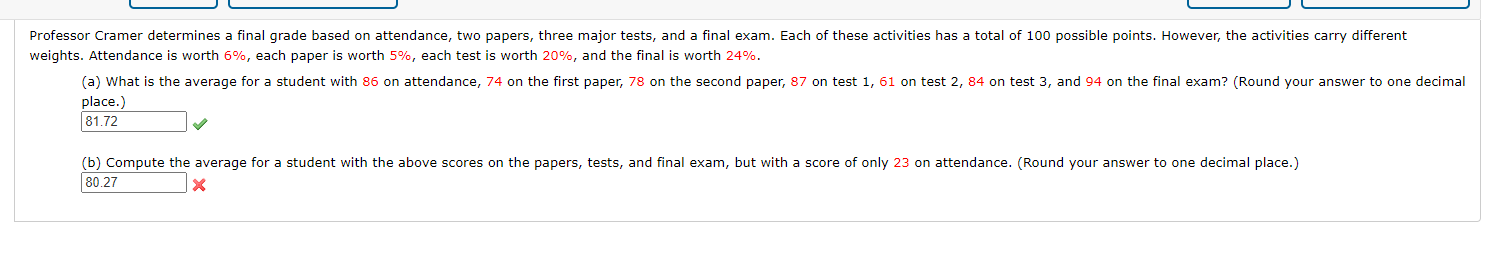The image is a cropped section from a webpage, focusing on a vertically narrow but horizontally wide rectangular box that spans the width of a computer screen. The box is outlined by a thin gray line and predominantly displays a blank white background. A light gray bar is positioned at the top of the box, featuring four search bars or buttons, though the text on them is indecipherable due to the limited view.

Inside this outlined box, there is detailed educational content in small black font, which becomes readable when zoomed in. It outlines Professor Kramer's grading criteria: attendance, two papers, three major tests, and the final exam, each worth a possible 100 points but weighted differently. The weights are as follows: attendance (6%), each paper (5%), each test (20%), and the final exam (24%). The weights are visually distinguished by their red color, contrasting with the black color of the rest of the text.

Following the grading criteria are two questions:

**Question A:**
- **Task:** Calculate the average for a student with the following scores: 86 (attendance), 74 (first paper), 78 (second paper), 87 (test 1), 61 (test 2), 84 (test 3), and 94 (final exam). The instruction includes rounding the answer to one decimal place.
- **Answer Provided:** 81.72
- **Feedback:** A green checkmark indicates the correctness of this answer.

**Question B:**
- **Task:** Compute the average for the same student scores as specified in the first question but with a different attendance score of 23. The instruction also includes rounding the answer to one decimal place.
- **Answer Provided:** 80.27
- **Feedback:** A red X signifies that this answer is incorrect.

The structure of the box and the interactive nature of the answers suggest that this is an online test interface. The detailed depiction of both questions and the vibrant use of red for specific numbers effectively highlight important elements for the students.